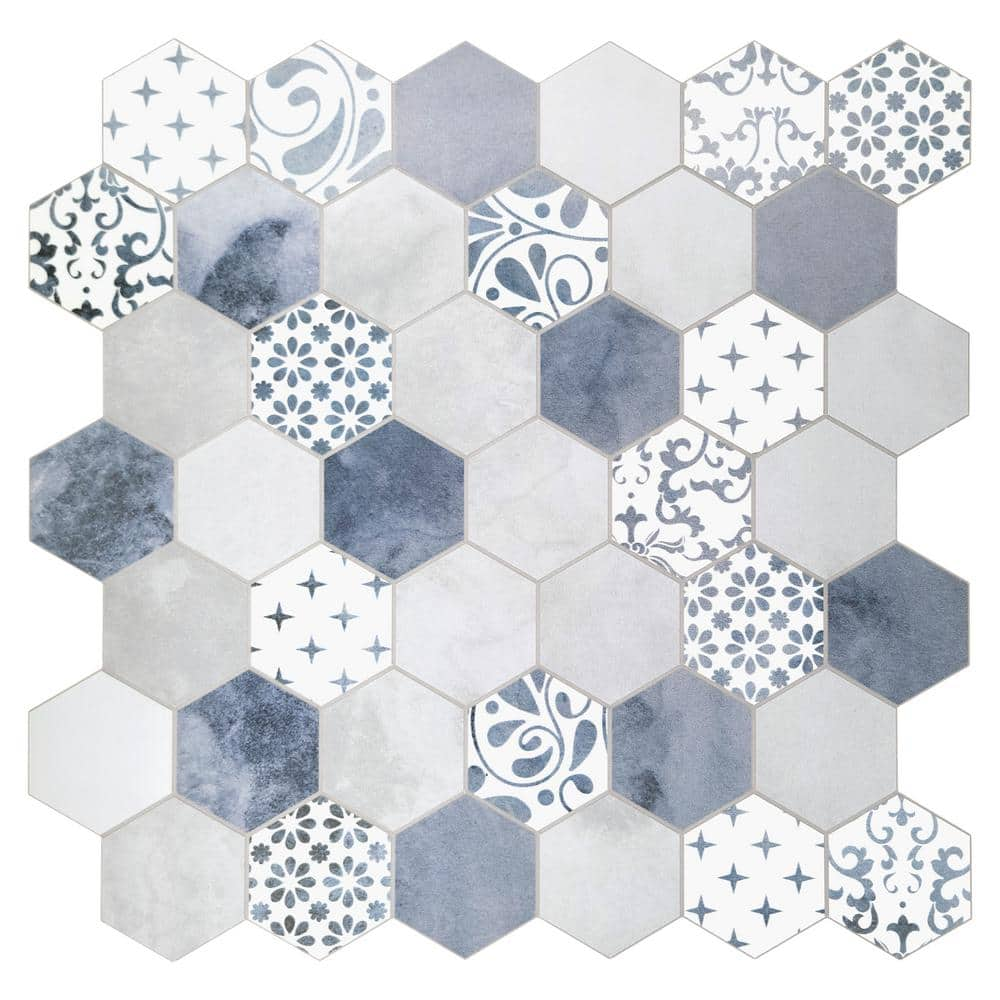The image depicts a tessellation of hexagonal tiles arranged in a meticulous pattern without any gaps between them. Spanning seven rows of six tiles each, the mosaic showcases a diverse palette of shades, including various grays, dark blues, and whites. The tiles feature a mix of plain colors and intricate designs, such as white tiles adorned with dark blue stars, blue argyle flowers, and blue floral prints. Some tiles display dark grayish-blue filigree patterns or multicolored gradients of gray, creating a harmonious yet complex visual interplay. The overall layout has a slightly jagged border due to the hexagonal shape, and the tiles are separated with a gray grout. This detailed and repetitive pattern could seamlessly fit into a floor space within a home, offering both aesthetic appeal and intricate design.